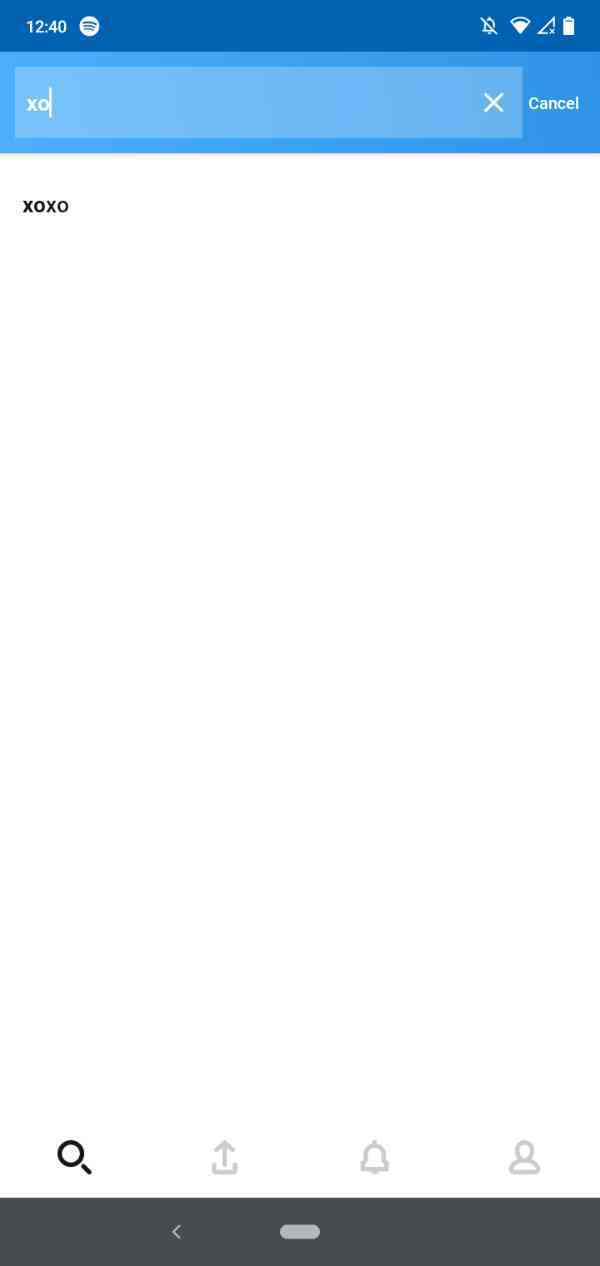The image is a screenshot taken on a phone or tablet, featuring an interface with predominantly white elements against blue and gray backgrounds. At the very top, there is a dark blue header displaying the time (12:40) on the left, along with a circular icon featuring lines. On the right side of this header, four icons are visible, including those representing Wi-Fi and battery status. Below this header is a lighter blue section that contains an even lighter blue search bar. This search bar has 'XO' typed in white and includes a white 'X' and 'cancel' option on the right side.

Beneath the search bar, 'XOXO' is printed on the remaining white background of the screen, which remains empty until the bottom section. The bottom of the screen hosts four icons above a gray bottom bar: a magnifying glass for search, an upload or send button, a notification button, and a user profile button. Finally, the dark gray bar at the very bottom features a caret pointing to the left and a small circular rectangle centered within the bar.